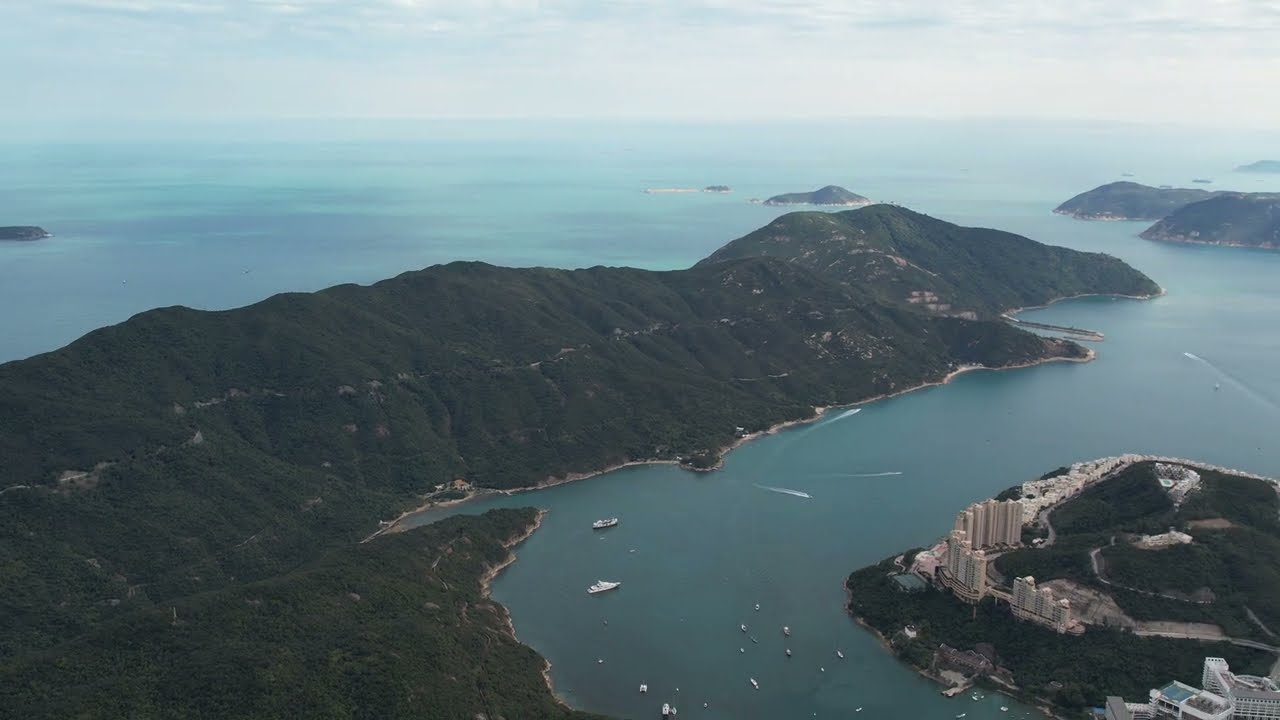This high-angle shot, potentially captured by a drone, helicopter, or plane, provides a sweeping view of a lush, mountainous coastal region dotted with islands. The landscape features dramatic, green-covered rocky outcroppings and smaller islets, all encircled by ocean waters. An inlet hosts several boats, some appearing to be sizable yachts while others resemble fishing vessels or speed boats leaving trails behind. In the bottom right corner, a prominent outcropping of land extends into the inlet, lined with tall, white skyscraper-like structures, likely hotels or casinos, indicating a tourist hotspot. Smaller buildings are scattered along the shoreline, connected by winding roads that traverse the steep, foliage-covered hills. The scene is bathed in an overcast light, with muted colors suggesting either a cloudy day or dusk, adding to the tranquil yet dynamic atmosphere of this coastal haven.